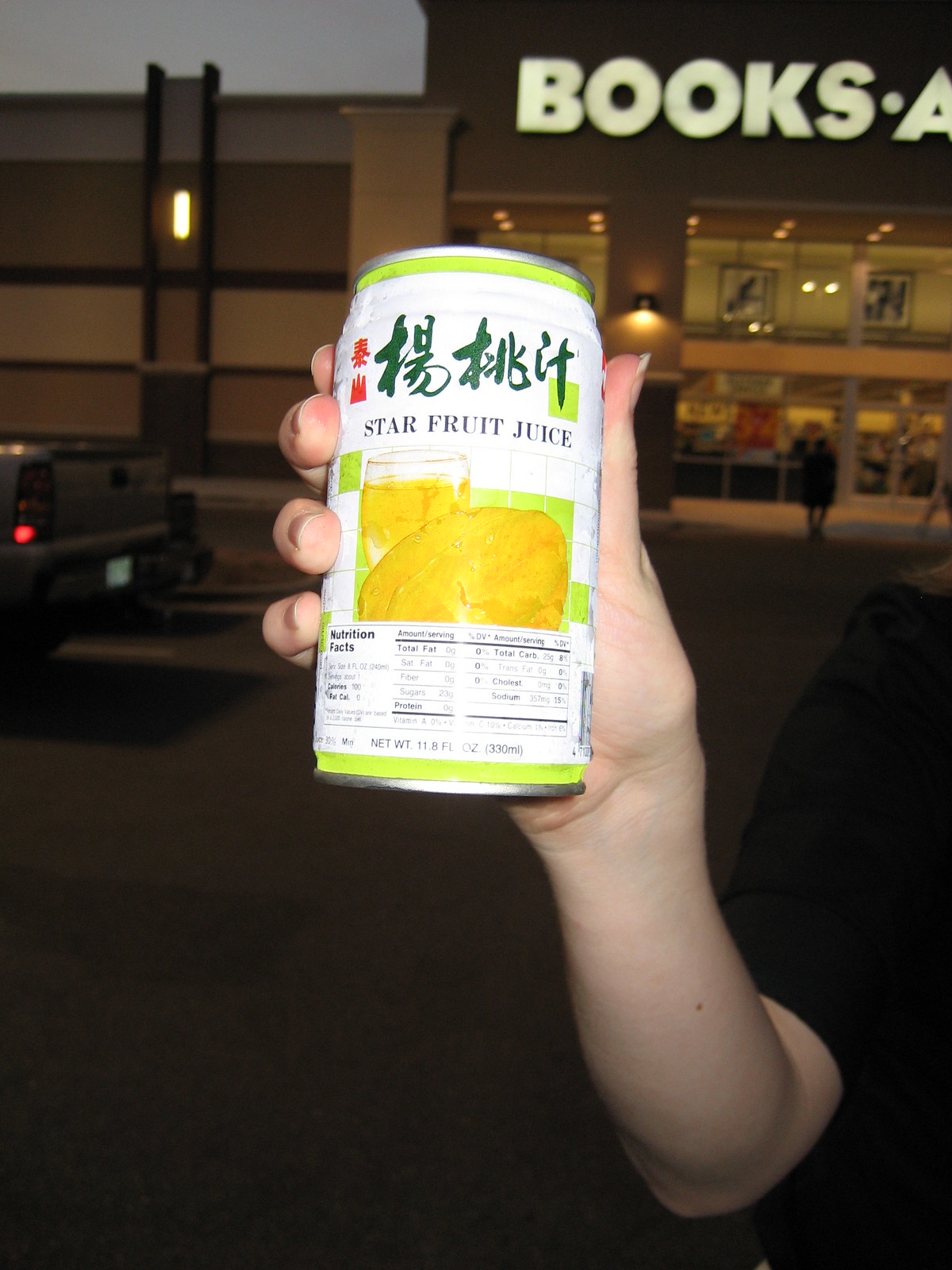In this photograph, a person holds a white can of beverage in their right hand, positioned centrally in the image. The can features lime green rims at the top and bottom, with dark green lettering across the center in a non-English script, and below that, it reads "Starfruit Juice" in the same color. Accompanying the text is an image of the starfruit juice itself. The setting is a parking lot outside a large plaza store, with the illuminated sign partially reading "Books and something." It is dusk, with the sky dimly lit as the sun has just set but it isn’t completely dark yet. On the left side of the image, some cars are visible in the parking lot, contributing to the ambient, early evening atmosphere.